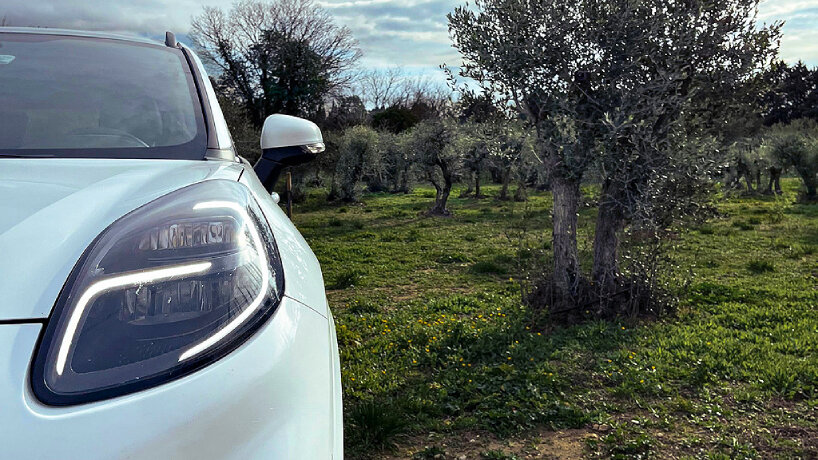In this evocative image, the left side prominently features the striking front half of a white Porsche facing the viewer. The vehicle’s headlight, half of the hood, bumper, and front windshield are clearly visible, along with a portion of the side window that boasts a sleek black trim. The right side of the picture contrasts sharply with the car, showcasing a lush carpet of grass interspersed with tiny, vibrant yellow flowers. Dominating the foreground is an ancient, gnarled tree, while the background reveals a grove of similarly aged trees, their barren branches and grayish hue giving them an almost ghostly appearance. Above, the sky is adorned with drifting clouds, with a particularly dark, foreboding cluster situated in the top-left corner, adding an element of drama to the serene yet haunting landscape.